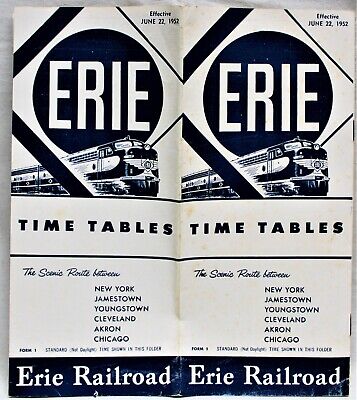The image features two identical Erie Railroad brochures side by side, set against a gray background. Each brochure prominently displays the text "Effective June 22, 1952" in the top right corner. Below this date, the word "ERIE" is spelled out in white letters within a dark blue circle. Immediately beneath the "ERIE" label, a detailed illustration of a train is featured. Following this, the brochures list "Timetables," succeeded by italicized text. The places "New York, Jamestown, Youngstown, Cleveland, Akron, Chicago" are highlighted next. At the very bottom of each brochure, "Erie Railroad" is clearly written. Overall, these brochures emphasize the key stops and effective date for the Erie Railroad's timetables.